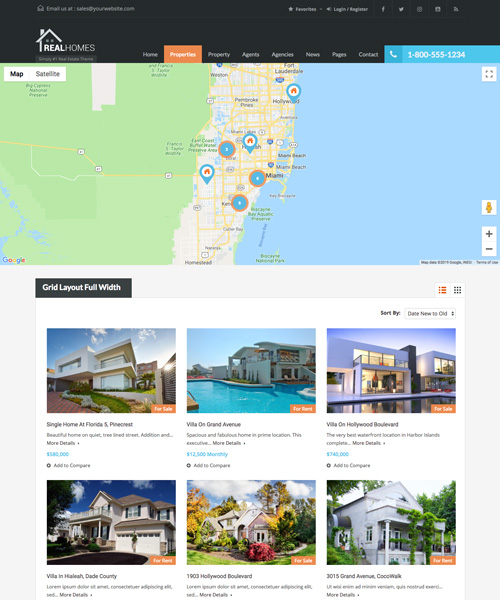The image captures a sophisticated real estate website. In the top left corner, the white text "Real Homes" stands out against a black background. To the right of this logo, a navigation bar features tabs for "Home," "Properties," "Property Agents," "Agencies," "News," "Pages," and "Contacts." The contact number, prominently displayed in bold white text on a blue background, reads 1-800-555-1234, situated at the top right.

The highlighted "Properties" tab is marked with an eye-catching orange color, leading to the main content area. A centered map is displayed, and just below it, the text "Grid Layout Full Width" is noted. Six property listings are laid out in a grid format.

The first property, located in the top left, is listed as a "Single Home at Florida." This beautiful home, situated on a quiet, tree-lined street, is priced at $580,000. The price appears in blue text while the description is in black.

To its right, the second property on "Grand Avenue" is available for a monthly rent of $12,400. This listing highlights a house with a blue swimming pool against a backdrop of a white exterior.

The third property on the top right is a villa located on Hollywood Boulevard, up for sale at $360,000.

In the bottom left, another villa is listed for rent in a location described as "left-hand country."

Centrally located at the bottom, a property at "900 Hollywood Boulevard" is also marked for sale, although its price is not shown.

Lastly, the bottom right features a white house with green trees, situated at "315 Grand Avenue, Cookwork," available for rent.